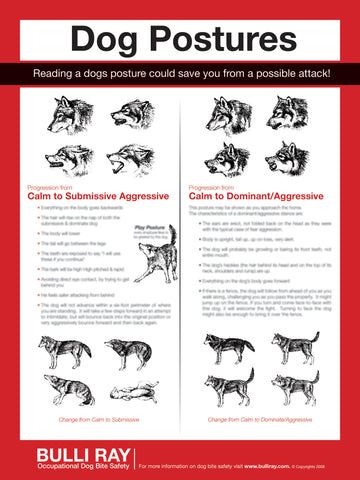This vertically aligned rectangular poster features a red border framing a white background. At the top, "Dog Postures" is prominently displayed in black print against a white rectangle. Beneath the title, a bold statement reads, "Reading a dog's posture could save you from a possible attack," in white print on a black background strip. The poster is divided into four sections showcasing dog illustrations, likely of breeds resembling German Shepherds or Huskies, demonstrating various expressions and postures.

In the upper left section, four close-up images of the dog's face transition from neutral to angry. The upper right mirrors this with another set of four facial expressions. Below, the lower left section presents four full-body images of a dog in submissive positions, including one on its back with legs up. The lower right section displays four full-body images of a dog in dominant stances. 

The center of the poster is divided by two main headings in red. On the left, "Progression from Calm to Submissive-Aggressive" includes multiple bullet points detailing the text in black print. On the right, the heading reads "Progression from Calm to Dominant-Aggressive," also with several bullet points and accompanying detailed descriptions. At the bottom, the creator's name, "Bully Ray," is written in large white letters.